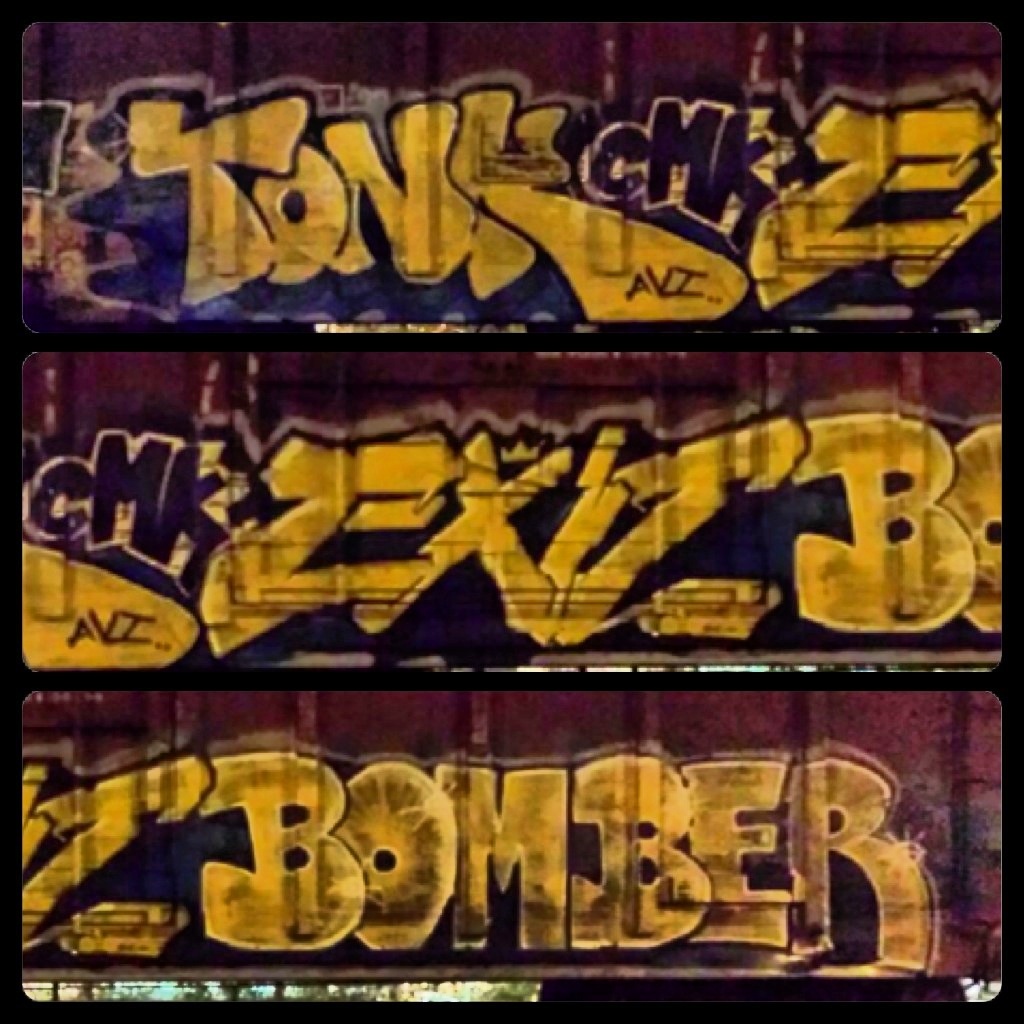The image features a collage of three sections of graffiti on the side of rusted, brown train cars, each separated by a black border. The vibrant graffiti is set against this background. In the first section: bold, stylized yellow letters spell out "Tony CMKZ," with "CMK" rendered in smaller, black text, illuminated by a white outline and accented with blue infill to make the yellow stand out. Additionally, within the Y of "Tony," the initials "AVI" can be found. The second section continues seamlessly from the first, with "EX" from the previous "Z" leading into "EX is," again featuring the recurring "CMK." The third and final section completes the message with "B.O.M.B.E.R.," suggesting the full statement reads, "Tony CMK Zex is a bomber." The background suggests an industrial or urban setting, possibly a train yard, enhancing the gritty authenticity of the artwork.